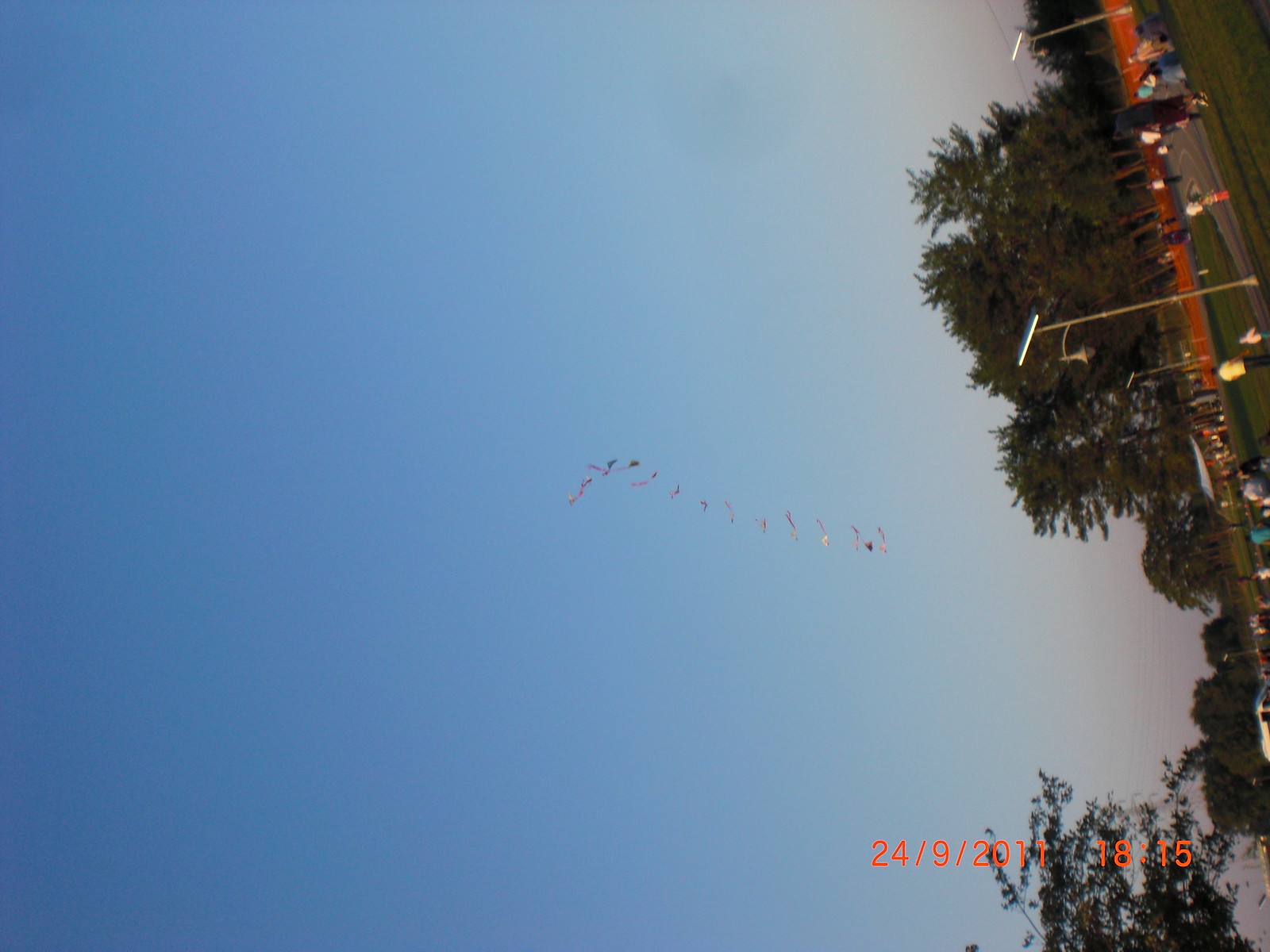This image appears to have been taken accidentally in a sideways orientation. The horizon line runs perpendicular across the photo, slightly out of focus. Dominating the frame is a predominantly blue sky, which lightens near the meeting point with an orange wall and tree line towards the right side. Scattered figures, perhaps around 20, occupy a wide pavement area, suggesting a park-like landscape. Among the detailed elements is a faint line of approximately 12 birds flying in a straight pattern through the sky, centrally positioned. Grass and concrete paths are visible, contributing to the park ambiance. Notably, a date and time mark in red letters—24-9-2011 18:15—appears at the bottom, indicating it was captured with a digital camera.